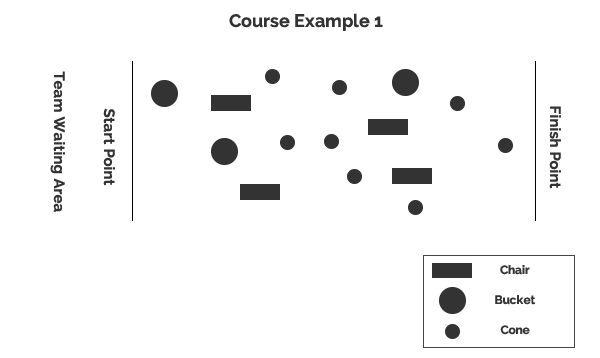This black-and-white image appears to be a textbook-style diagram of an overhead view of an obstacle course. It is labeled at the top as "Course Example 1." The left side has the label "Starting Point/Team Waiting Area," while the right side is marked as "Finish Point." These two points are connected by lines that the course participants presumably follow. Inside the course area, there are a series of solid black shapes: 11 circles and 4 squares. According to the legend located within a thin-lined square at the bottom right corner, rectangles symbolize chairs, large circles stand for buckets, and smaller circles represent cones. The course layout includes four chairs, three buckets, and eight cones, all arranged in no particular order.